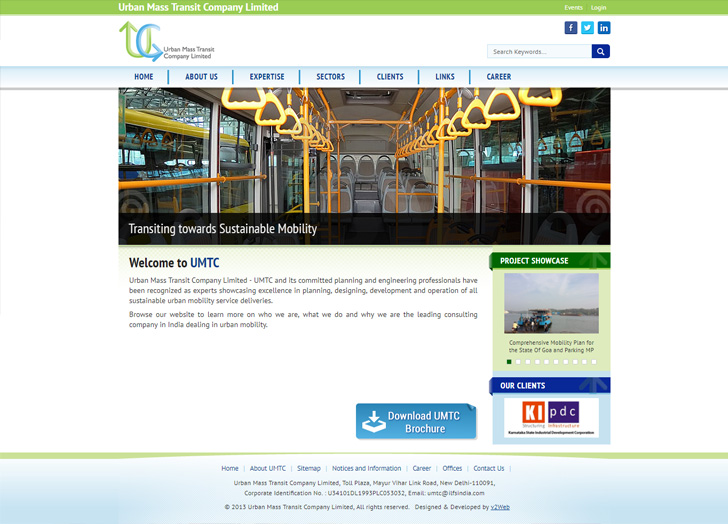The screenshot captures the homepage of the Urban Mass Transit Company Limited's website displayed on a computer monitor. At the top of the page, a lime green banner extends across the screen, featuring bold white text on the upper left that reads "Urban Mass Transit Company Limited." On the far right of this banner, the words "Events" and "Login" appear in white as well, accompanied by three social media icons for Facebook, Twitter, and Instagram positioned below these links.

Directly beneath this banner, a white rectangular section displays the company's logo: a green "U" with a blue "C" overlaid on it. To the right of the logo, "Urban Mass Transit Company Limited" is written in black lettering. On the far right of this section is a search box with a magnifying glass icon.

Below this section, a light blue menu bar features navigation labels in dark blue, separated by vertical blue lines: "Home," "About Us," "Expertise," "Sectors," "Clients," "Links," and "Career."

The primary graphic at the top of the page, situated under the banner, depicts the interior of a city bus. The image captures a view down the aisle toward the rear of the bus, showcasing yellow overhead handles and multiple seats.

At the bottom of this graphic, a black rectangular area has white text on the left saying "Transiting Towards Sustainable Mobility." Below, in a white section, the phrase "Welcome to UMTC" is prominently displayed followed by a brief paragraph of descriptive text in black.

On the right side of the page, a small, slightly blurry image of people in a boat on water is labeled "Project Showcase" in white text set against a dark green banner.

The very bottom of the section features a blue banner with white text that reads "Our Clients." Below this, a section highlights an orange square with "KI" in white and a blue square with "PDC" in white. To the left, the text "Download UMTC Brochure" is presented in blue and white. A horizontal green line divides the section from the footer.

The footer includes typical website links displayed in blue: "Home," "About UMTC," "Sitemap," "Notices and Information," "Career," "Offices," and "Contact Us."